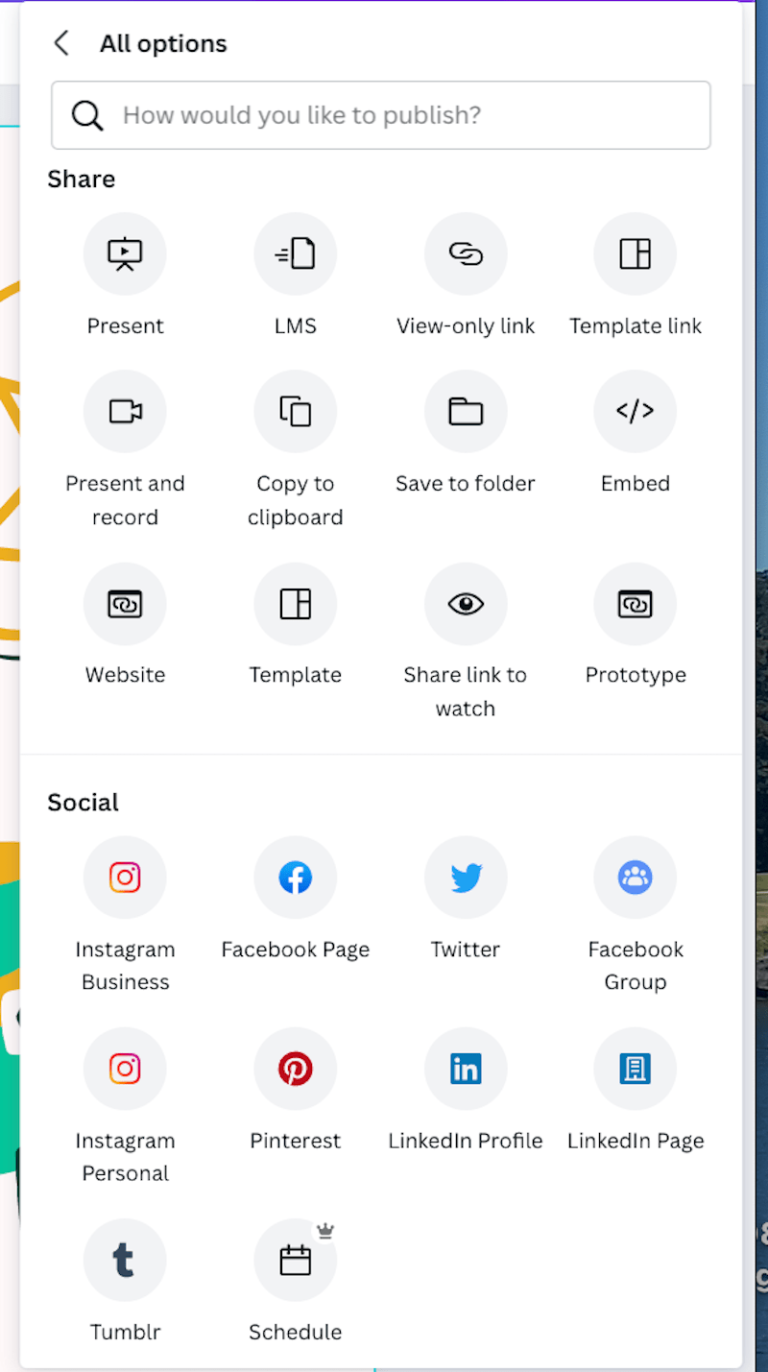Screenshot of a User Interface for Publishing and Sharing Content:

The screenshot showcases a user interface designed for publishing and sharing content, titled "All Options" at the top. It features a search box pre-populated with the query "How would you like to publish?". The interface is divided into two main categories: "Share" and "Social".

Under the "Share" category, various options are listed:
- Present
- LMS (Learning Management System)
- View Only Link
- Template Link
- Embed
- Save to Folder
- Copy to Clipboard
- Present and Record
- Website
- Template
- Share Link to Watch
- Prototype

Beneath the "Social" category, the available platforms for sharing are displayed:
- Instagram Business
- Facebook Page
- Twitter
- Facebook Group
- Instagram Personal
- Pinterest
- LinkedIn Profile
- LinkedIn Page
- Tumblr
- Schedule

Users must select how they want to publish their content and decide on the appropriate audience and method for sharing across the various social networks provided at the bottom of the screen.